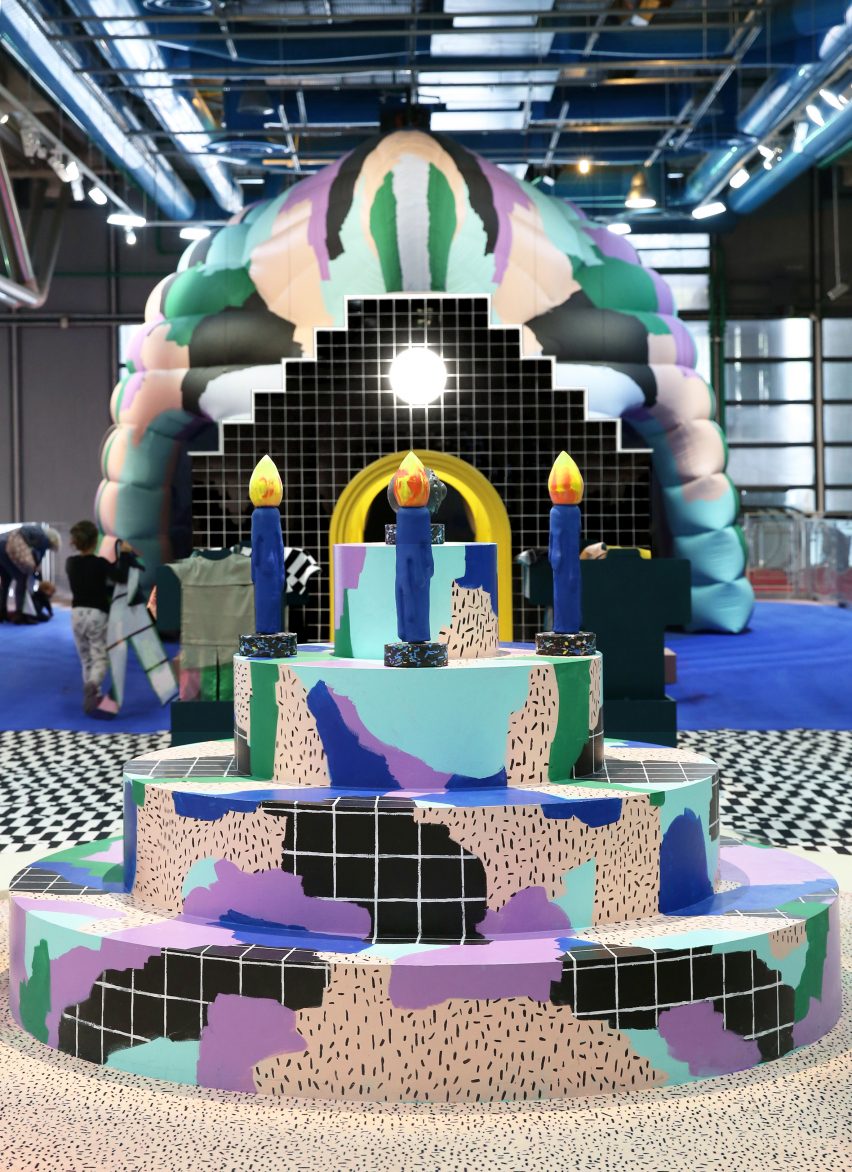The image shows an indoor scene with a high ceiling supported by metal rafters and hanging lights. The floor features a white surface with speckled black patterns, creating a distinct backdrop for the centerpiece: an elaborate, fake, four-tiered cake-like sculpture. This sculpture, positioned centrally in the frame, has four circular tiers that diminish in size from bottom to top. Each tier is decorated with an intricate mix of patterns, including black and white checkerboard tiles, black dots on a whitish cream and pink background, and vibrant splashes of purple, blue, and green. Notably, the third tier prominently displays three large blue candles with yellow-orange flames crafted to look as if they’re burning.

In the background, there is a black tiled wall with white grout, contributing to the visual texture of the room. Adding to the dynamic atmosphere, a semi-circular inflatable mountain with a black grid pattern and multicolored splotches (purple, blue, green) hangs above. Some children are visible in the distant background, indicating the setting might be an interactive exhibit or an art installation. Overall, the image captures a creative fusion of art, playful design, and whimsical elements within what appears to be an art gallery or exhibit space.